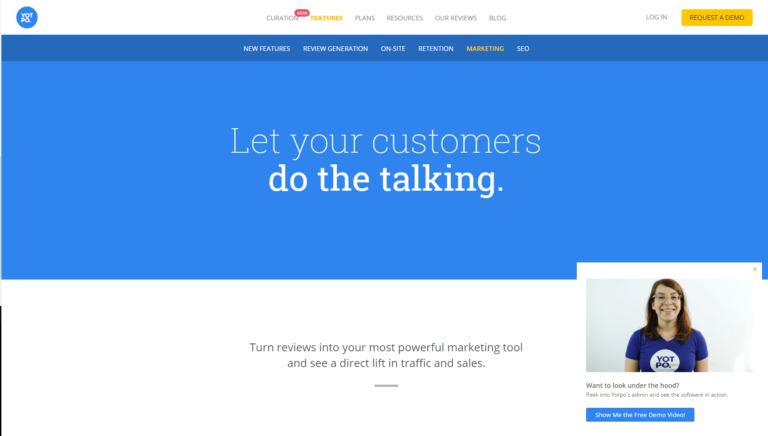This image is a screenshot of a website featuring a prominent call-to-action in the middle. The central area is highlighted with a royal blue background, showcasing the message "Let Your Customers Do the Talking." Within this statement, the words "Do the Talking" are bolded and appear in a brighter white, emphasizing the action. Below this blue section, a white area contains the text, "Turn reviews into your most powerful marketing tool and see a direct link in traffic and sales," printed in black. A thin horizontal line, either green or gray, is positioned underneath this text.

On the right side of the image, there is a picture of a woman. She is dressed in a navy blue shirt that has a white circle with the text "Vat Po" inside it. She wears glasses and has shoulder-length brownish hair. Beneath her picture, there is a clickable box labeled "Show Me the Free Demo Videos." Additionally, a black text statement reads, "Want to look under the hood? Peek into your Yotpo's admin and see the software in action." The layout appears to encourage user engagement and exploration of the website’s offerings.